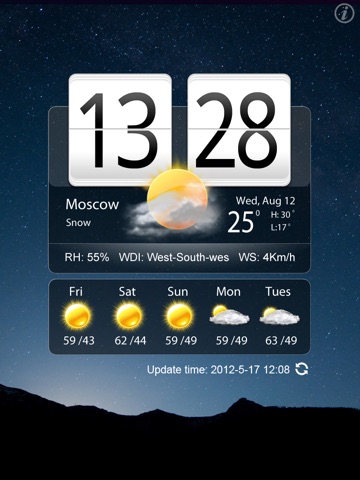The image depicts a nighttime scene, characterized by dark black mountains at the bottom, set against a navy blue sky dotted with white stars. 

On the left-hand side of the image, there is a light source whose nature is ambiguous — it appears to be either rising or setting. Above this light source, white text displays the date "2012/5/17" and the time "12:08."

There is a dark, transparent rectangular overlay featuring the abbreviated days of the week — Friday (Fri), Saturday (Sat), Sunday (Sun), Monday (Mon), and Tuesday (Tue). Icons within this overlay indicate that both Friday and Saturday will be sunny, while Sunday, Monday, and Tuesday will experience a mix of sun and clouds. On the left side of this rectangle, white text lists temperature ranges: "59/43," "62/44," "59/49," "59/49," and "63/49."

Below this, another smaller transparent rectangle displays additional details: "RH: 55%," "WDI: west-south-west," and "WS: 4KM/H." Above this information, the text "Moscow snow" appears alongside more icons illustrating a mix of sun and clouds. The date for this forecast is specified as "WED, August 12th, 25," with a high temperature of 30°C and a low of 17°C. The numbers "13" and "28" are also visible in black text, possibly denoting further details that are not explicitly decipherable.

Overall, the image effectively combines weather information with the serene aesthetics of a nighttime landscape.